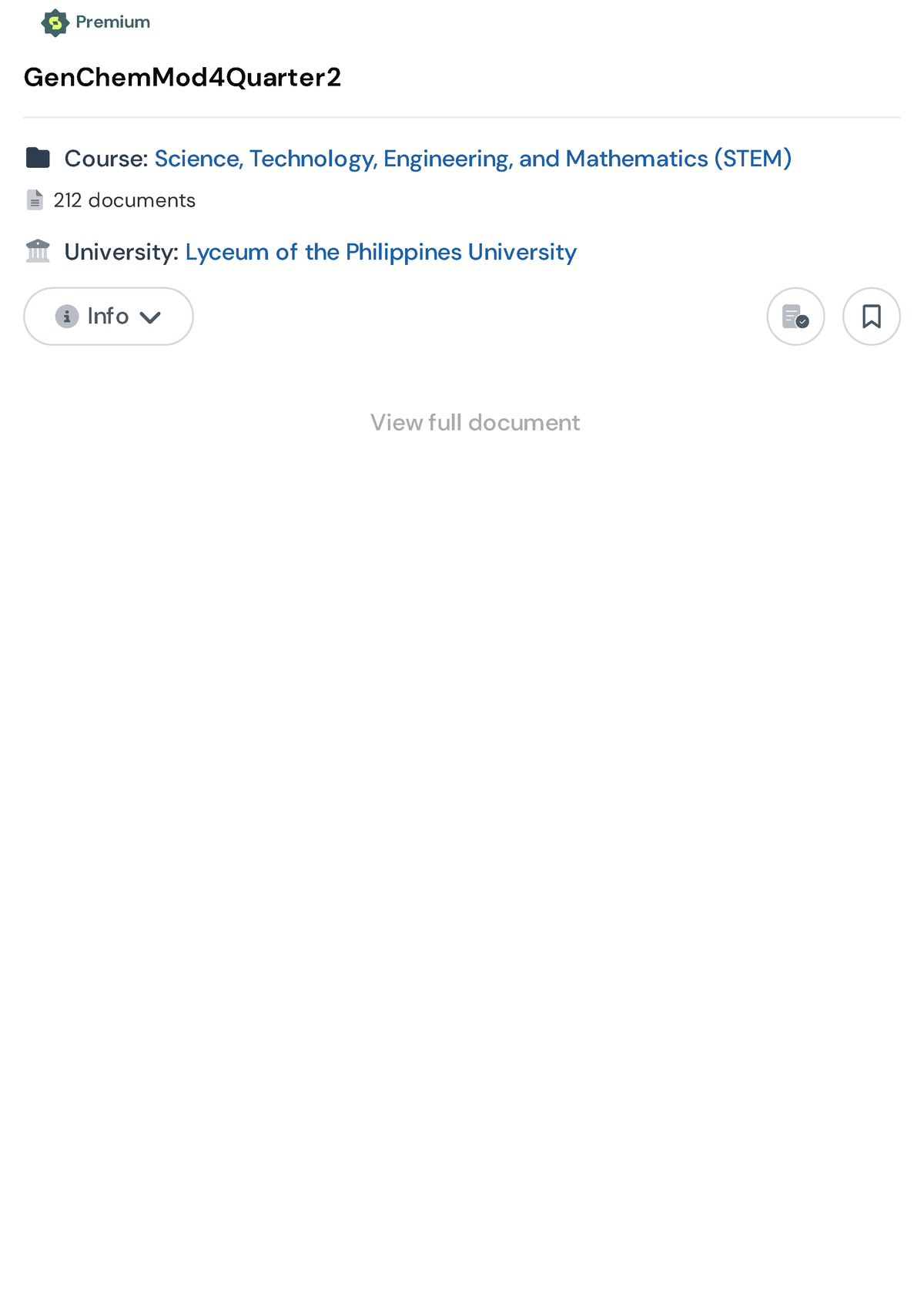This image appears to be a partial screenshot of a website. At the top, the word "Premium" is displayed next to a green, multi-pointed star-like icon with rounded points. Within this green star, there is another symbol, though its shape is indistinct.

Below this, the main title reads "Jen Kim Mod for Quarter Two," in bold black text. A thin, light line stretches across the width of the page immediately underneath the title. Adjacent to this title, there is a folder icon followed by the word "Course," which is then described as "Science, Technology, Energy, and Mathematics" in parentheses.

Further down, a document icon indicates "212 documents." An icon resembling a Roman-style building is accompanied by the word "University." Additionally, there is an icon representing the Philippines University. Below these, an information (info) button that triggers a drop-down menu is visible. On the opposite side of the page, there are buttons for bookmarks and what appears to be a page icon.